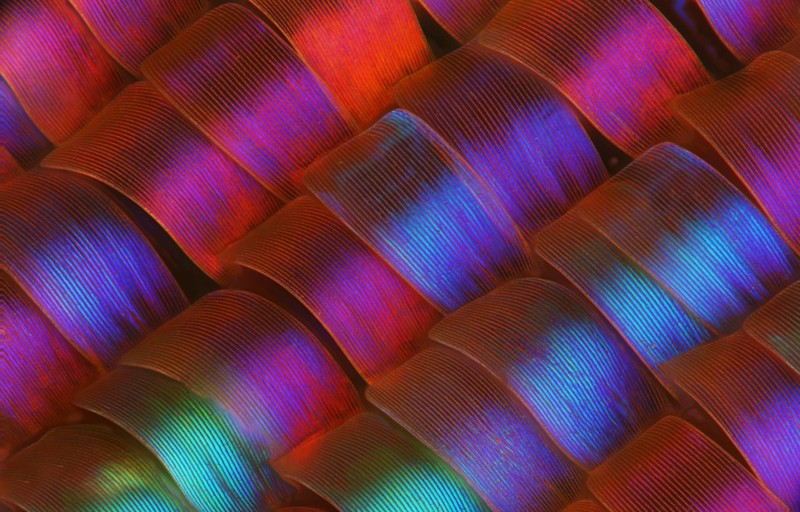The image displays a close-up view of an abstract material composed of rippled, scale-like arcs arranged in diagonal rows. These arced elements, resembling continuous loops of ribbon or tile, exhibit striations along their vertical axis, creating a textured surface. The ripples flow rhythmically from the bottom left to the upper right of the frame, echoing the wave-like pattern of a tile roof. The vibrant colors—ranging from bright pinks and greens to various shades of blues, purples, and deep reds—interact dynamically with the lighting. This combination of hues and the way the light hits the material gives it a glowing, almost metallic appearance, suggestive of being under a dark light or illuminated by sunlight. There are five distinct diagonal rows of these arches, adding to the complexity and allure of the visual.